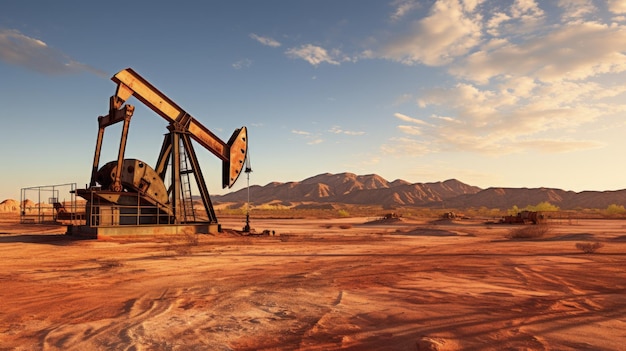The image depicts a vast desert landscape characterized by reddish and light brown soil stretching out under a clear, light blue sky. Scattered white clouds float on the far right, where the sunlight seems to be coming from, illuminating this side of the scene. Directly in front, a range of brown, slightly elevated mountains extends across the entire horizon, ending at the right edge of the picture. In the left side of the image stands a prominent yellow oil derrick surrounded by metallic tubes or fencing, with its nose directed towards the ground. Thin wires from the derrick are visible, suggesting its active involvement in drilling. Far off in the distance on the right, there is a hint of greenery, adding a touch of color to the otherwise arid setting. The scene is devoid of any human presence, emphasizing the isolation and vastness of the desert environment.